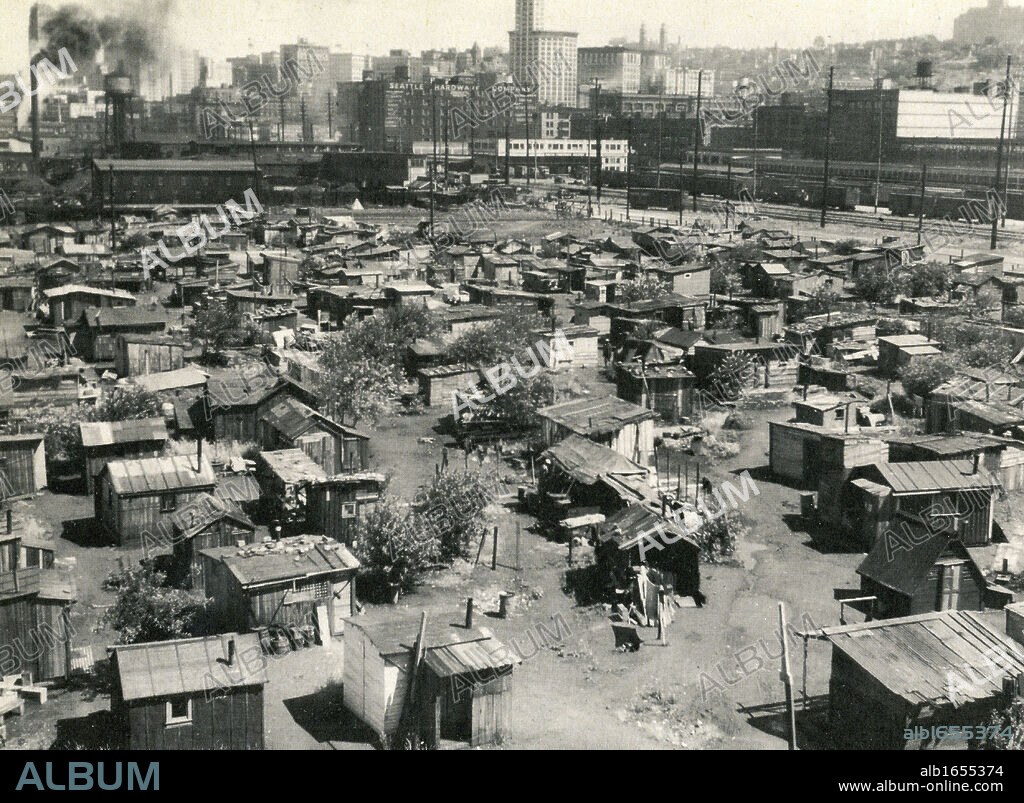This black and white aerial photograph, taken from a few stories high, captures a sprawling shantytown with an array of tiny, makeshift shacks scattered across a vast dirt lot. The scene is evocative of the Great Depression era, possibly depicting a Hooverville. Sparse bushes dot the barren landscape, which is enclosed by a tall chain-link fence. In the distant background, industrial city buildings rise above 10 stories, juxtaposed against the impoverished community in the foreground. The grainy, low-quality image also shows trucks or train cars on what may be a road or track. Few figures are visible, emphasizing the desolation. Overlays of the word "album" appear multiple times across the image, with varying transparency, and a URL, www.album.online.com, is overlaid in the lower left corner.